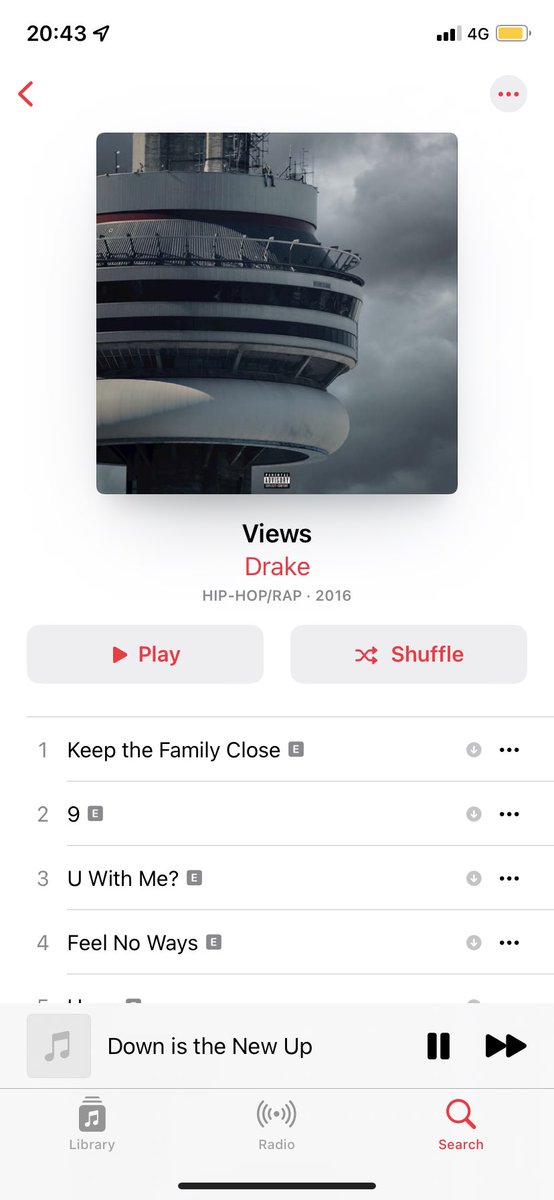A detailed caption for the image could be:

"The image displays a music app on an iPhone or Apple device with a white background. In the top left corner, there is a red back button, and in the top right corner, a red horizontal three-dot menu icon. Dominating the center of the screen is an album cover featuring grey clouds and a grey and slightly white building. The album cover includes a black 'Advisory' label at the bottom. Centrally, the album title 'Views' is displayed and beneath it, the artist's name 'Drake' is written in red. It also indicates the genre 'Hip Hop/Rap' and the release year '2016.' Below this information, there are two grey buttons with red text: 'Play' on the left and 'Shuffle' on the right.

The tracklist shows four song titles: 
1. Keep the Family Close
2. Nine
3. You With Me?
4. Feel No Ways

There is a fifth song partially visible at the bottom. Beneath the tracklist, there's a currently playing song indicated as 'Down is the new app.' At the very bottom of the screen, three buttons are arranged: 'Left Bradley' on the bottom left, 'Radio' in the center, and 'Search' on the bottom right. The 'Search' button is highlighted in red, while the other two are grey."